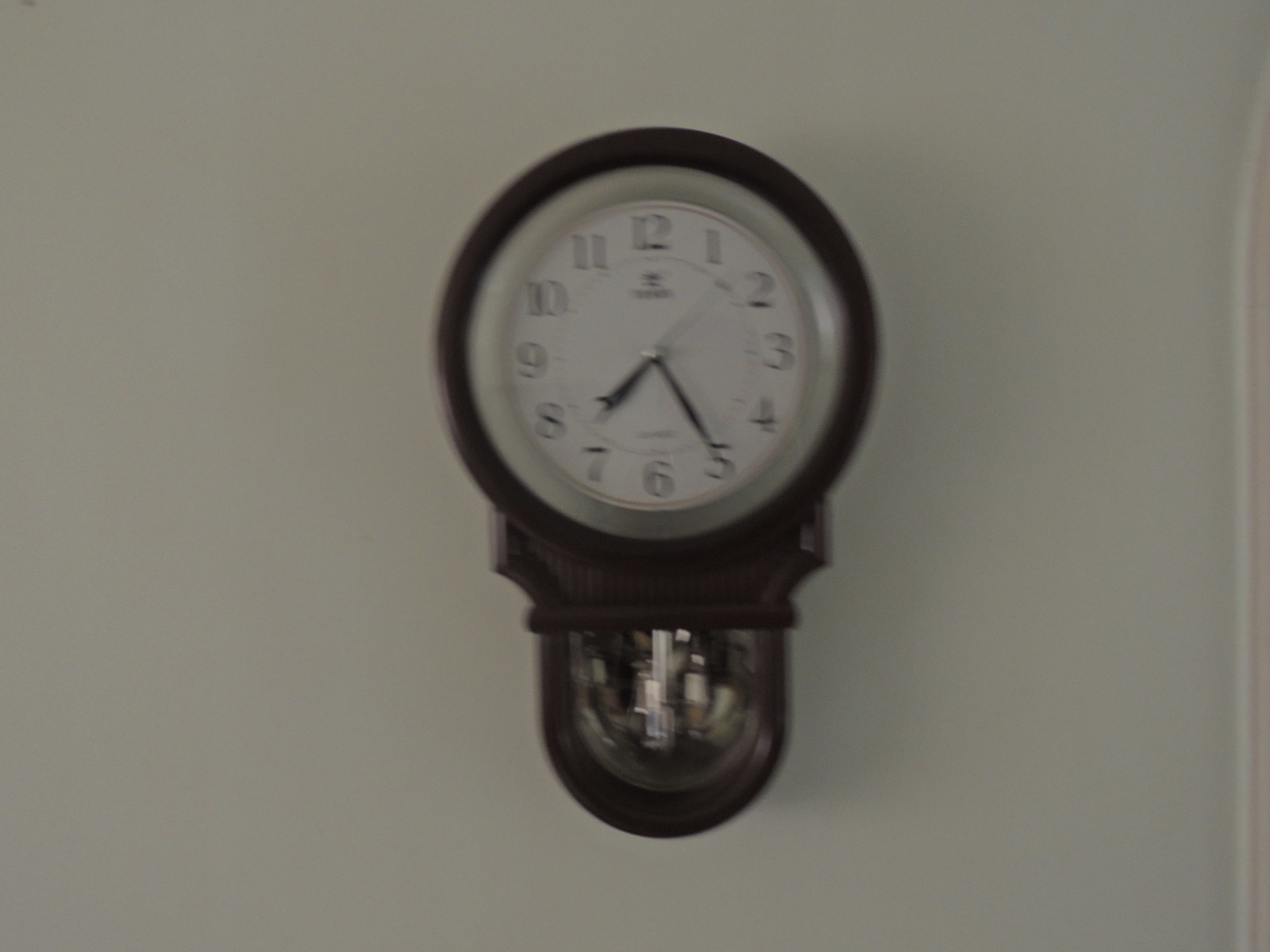This is an image of a clock hanging on a smooth, white or off-white wall that is somewhat poorly lit. The clock itself features a large circular face with a black or dark brown frame. Inside this frame, a smaller circle with a light gray border houses the actual white clock face, which has a single thin line in a light red or light brown color running around its edge. The clock clearly shows black numbers from 1 to 12 and has black hour, minute, and second hands indicating the time as 7:25 and 8 seconds. Below the circular part of the clock, there is a semicircular section made of clear glass, which allows a view of some internal clock mechanisms, although the details are hard to make out. The clock has an antique appearance, and it appears that you can see some of the mechanical intricacies inside through the glass. There is text on the clock face under the 12 and above the 6, but it is too small to read. The photograph is realistic but slightly blurry, adding to the old-fashioned feel of the image.